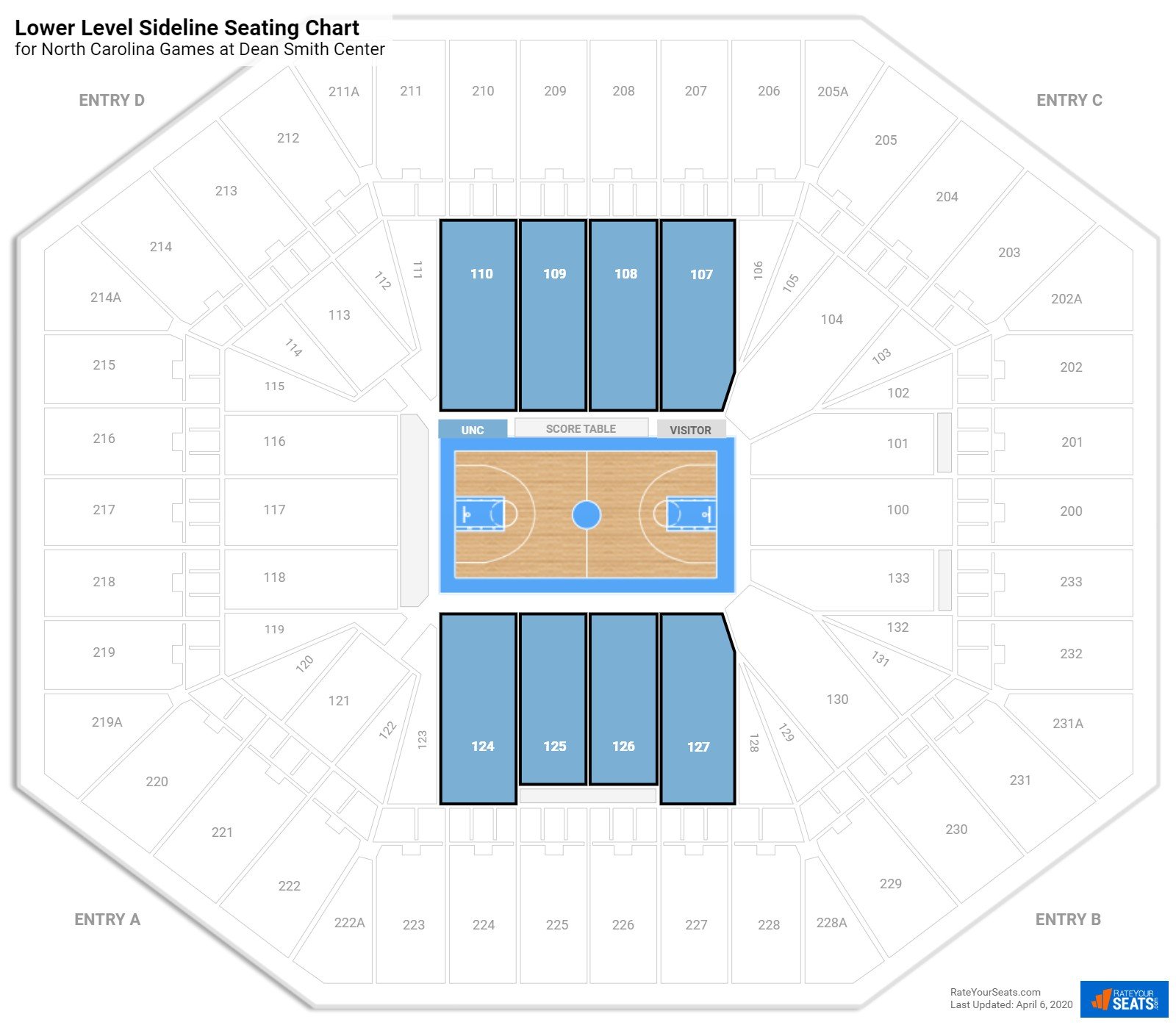This image depicts a detailed seating chart of the lower level sideline for a North Carolina basketball game at the Dean Smith Center. The chart features labeled entry points: Entry D at the top left, Entry C at the top right, Entry A at the bottom left, and Entry B at the bottom right. At the center of the image is the basketball court, surrounded by the available seating arrangements. Highlighted in blue are selected seats, specifically seats 107 to 110 and 124 to 127, indicating their chosen status. This visual guide serves to help attendees navigate and select their preferred seats for the game.